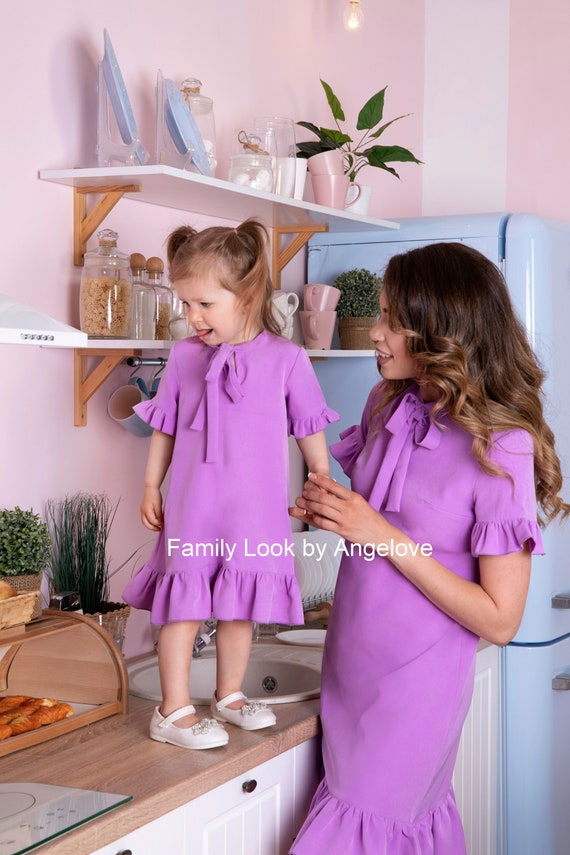This charming indoor photograph captures a heartwarming moment between a mother and her young daughter in a quaint, vintage-styled kitchen with pink walls and a light blue, old-fashioned refrigerator. The little girl, with her tongue playfully sticking out, stands on a light wooden countertop and is dressed in a silky, lilac purple dress. Her dress features ruffled short sleeves and a ruffled hem, with a bow tie around the neck. She sports white shoes with straps around her ankles. The woman standing next to her, presumably her mother, has long brown curly hair and wears an identical dress. They hold hands tenderly, sharing a matching, coordinated look. Behind them, a white ceramic sink is visible, alongside shelves that display coffee cups, planters, and various food items in canisters. A bread box containing bread sits on the counter. This delightful image with the overlay text "family look by angel love and love" captures the essence of familial love and joy in their cozy, retro-styled home.